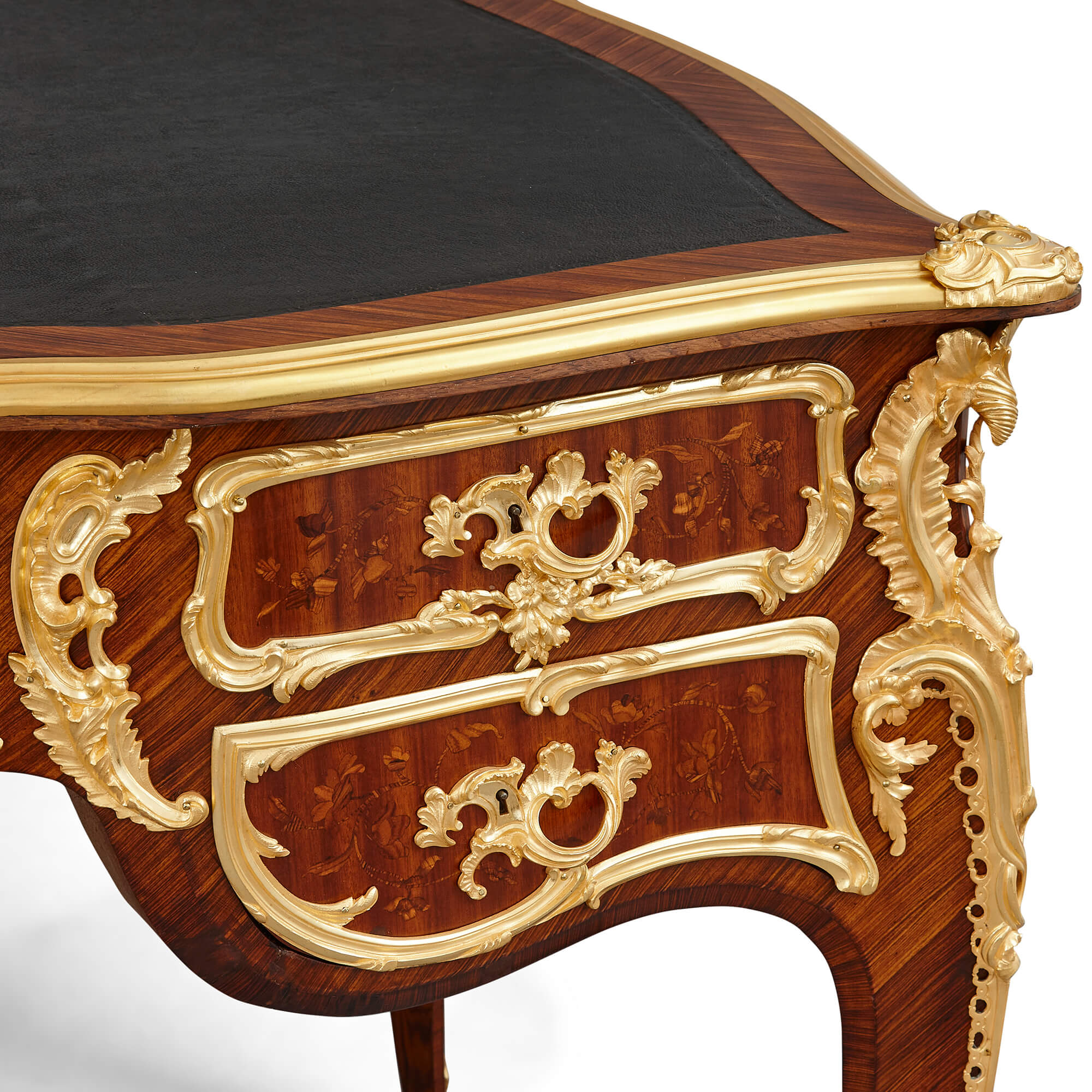This image features a close-up view of the corner of an intricate and ornate antique-style table, possibly a piano, showcasing a rich interplay of gold and dark wood. The table's edge is elegantly adorned with gold plating, which follows an intricate swirly pattern that resembles leaves, adding a touch of classical sophistication. This same gold detail is consistently seen around the outline where drawers would typically be, though these drawers appear non-functional due to the flush gold design against the dark, likely mahogany, wood. The top surface of the table is a solid flat black, framed by another rectangle of dark wood, emphasizing the antique elegance. The craftsmanship is meticulous, highlighting carved patterns and ornate gold trim work that stands against the deep, polished mahogany backdrop. This close-up angle elegantly captures the meticulous detail and craftsmanship involved while emphasizing the table's luxurious and vintage appeal.